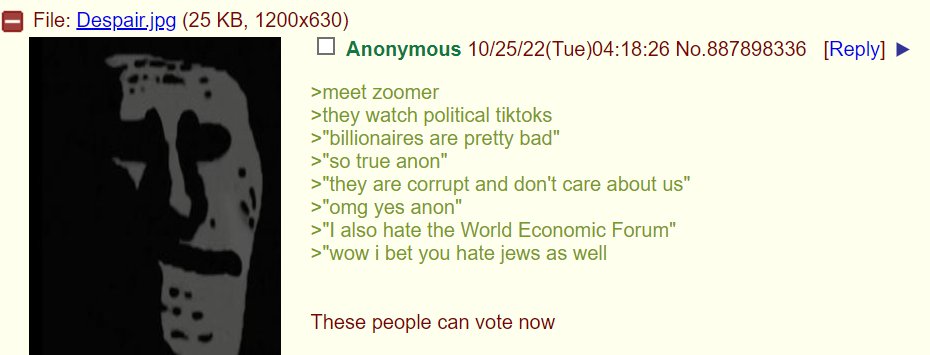**Caption:**

In this digital file, the background is a soft pale yellow. In the upper left corner, there is a red square featuring a white minus sign at its center. To the right of the square is the word "file" in red text, followed by the blue text "despair.jpg". Accompanying these words, in red text within parentheses, are the file details: "25 kilobytes, 1200 by 630."

Beneath this header, on the left, is a large, rectangular image primarily colored black, featuring a gray face resembling a hockey mask. To the right of this image, at the top, is a white square followed by the username "anonymous" in green text. Next to the username, in red text, is the date "10-25-22" and in parentheses "Tuesday", followed by the time "4-18-26". Below the time, the number "887898336" is written, and to the right of this, within parentheses, is the word "reply" with a directional arrow pointing to the right.

Below this information, the text continues in green: "meet Zoomer", followed by: "they watch political TikToks. Millionaires are pretty bad. So true, Anon. They are corrupt and don't care about us. OMG, yes, Anon. I also hate the World Economic Forum." Following this conversation, a new message appears in red text stating: "Wow, I bet you hate Jews as well." At the bottom of the text block, in red, it ominously declares: "these people can vote now."